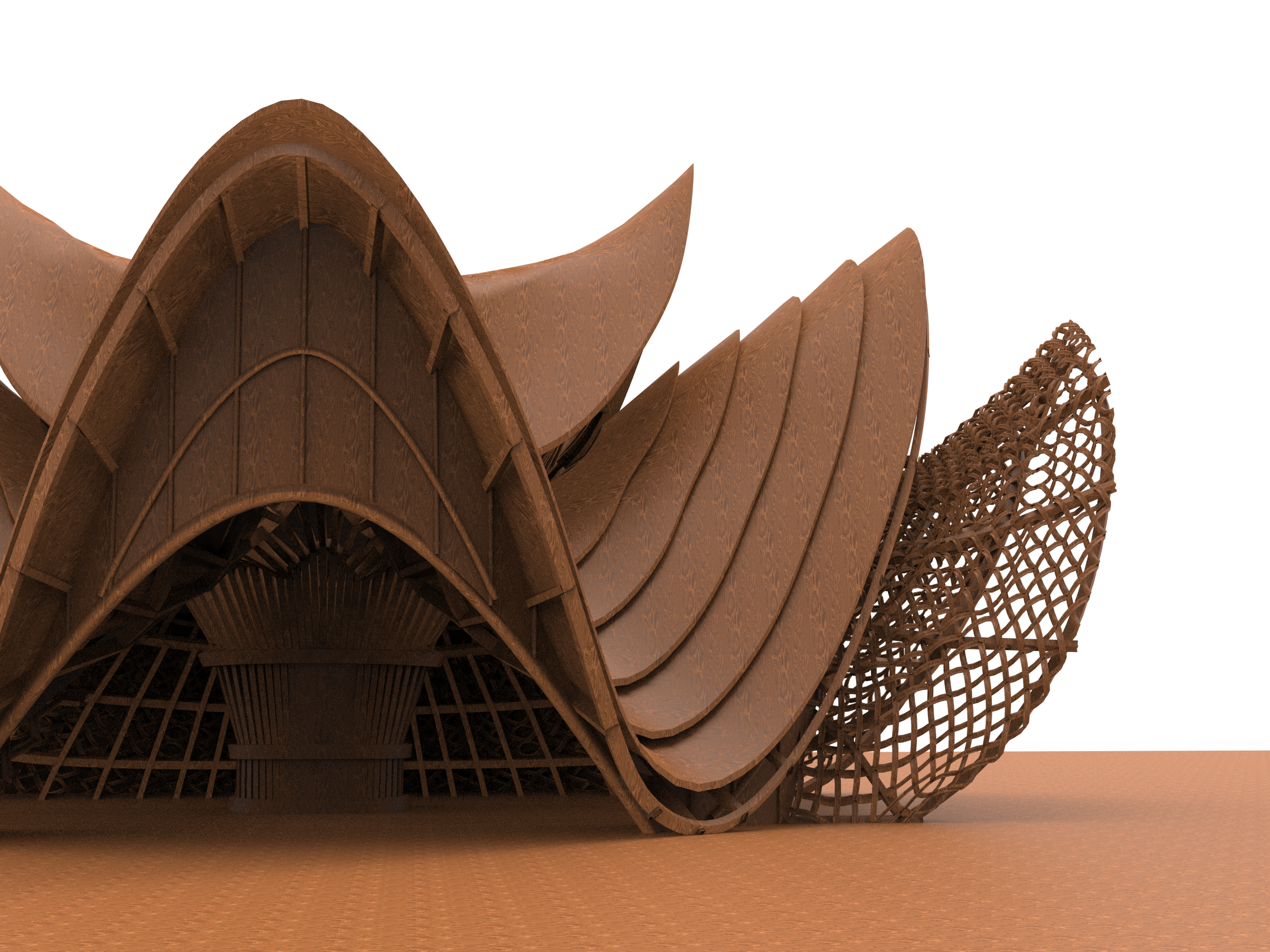The horizontal image showcases what appears to be a meticulously crafted model or computer-generated representation of an architectural structure or a sophisticated sculpture. Dominating the composition are numerous triangular, pyramid-like shapes that evoke a wave-like motion, reminiscent of the Sydney Opera House's iconic design but with taller and more angular peaks. These shapes, appearing to be made of a wooden material, sit elegantly on a medium brown table against a stark white background, enhancing their prominence. On the far right section of this intricate piece, the material transitions into a wicker texture, contrasting with the rest of the structure that appears to be solid cork wood. Intriguingly, within one of these undulating, wave-like forms, a visible bundle of straw is mounted, set against a wicker backdrop, adding an unexpected and organic element to the otherwise structural and geometric composition.